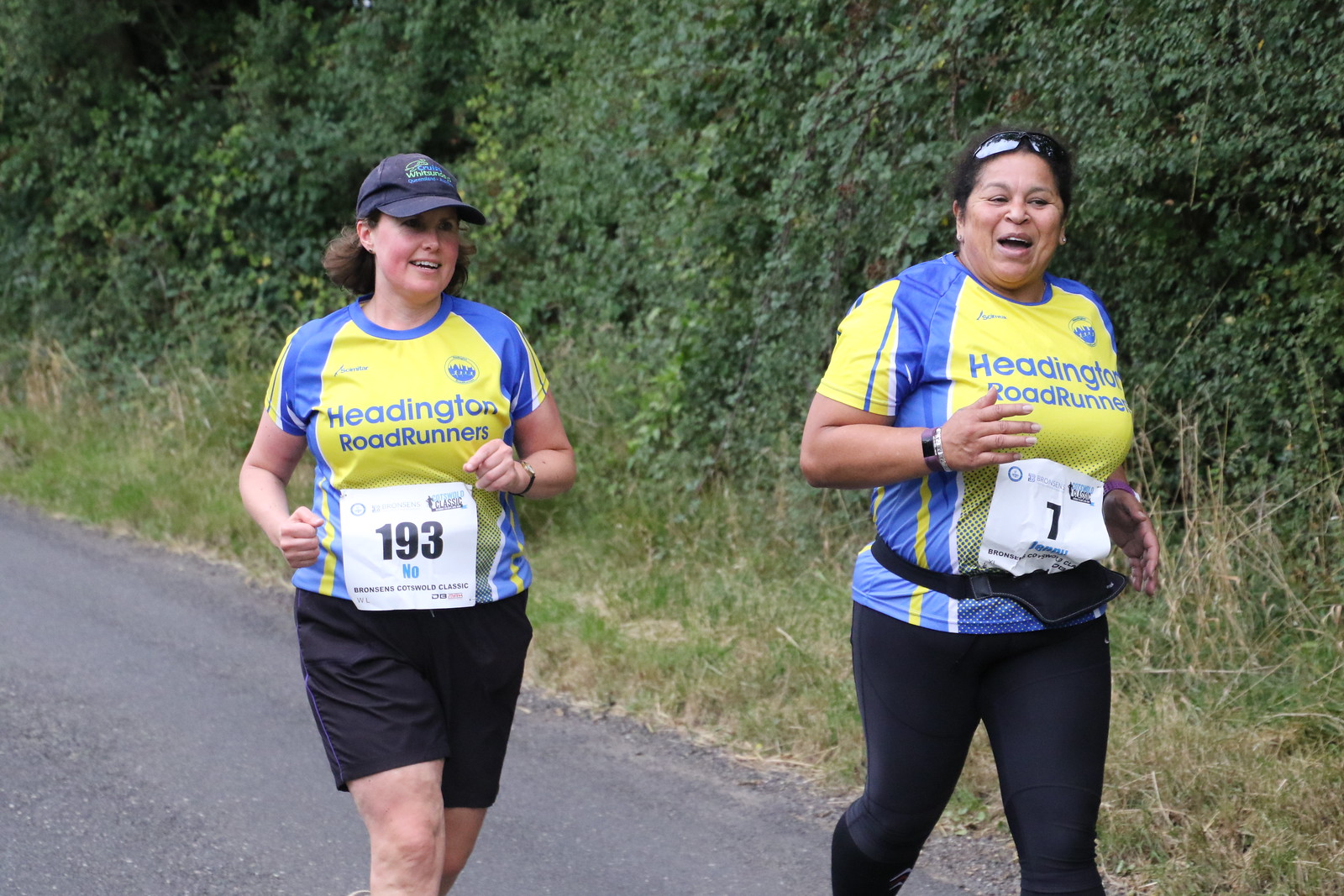This full-color daytime photograph captures two women running in a race on a paved road, surrounded by lush greenery, including trees, grass, bushes, and various plants. The woman in the lead appears to be Hispanic, with sunglasses propped on her head and wearing bib number 1. She is dressed in a Headington Road Runners club shirt and black tights. Just behind her, another woman, donning a hat and bib number 193, runs in a matching shirt and black shorts. Both women have their hands in a physical running motion, with one looking towards the camera and the other gazing straight ahead. Their vibrant yellow and blue boots add a pop of color to the dynamic scene.